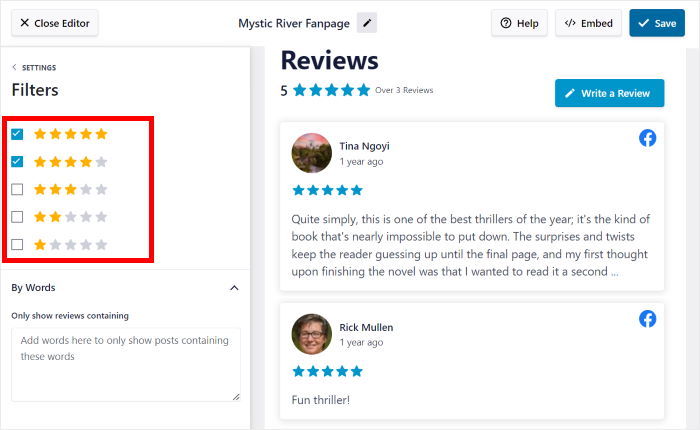The image showcases a reviews interface. In the top-left corner, there's a "Close Editor" button. To the left, a settings section is prominently displayed, with a focus on filters. A red square highlights the star rating options, specifically the selected five-star and four-star ratings. Below this, there is a section labeled "By Words," which includes an input box where users can type keywords to filter reviews that contain specific words.

On the right side, the reviews are shown. The first visible review is from Tina Ngoyi, who has given the book five stars. Her review reads: "This is one of the best thrillers of the year. It's the kind of book that is nearly impossible to put down. The surprises and twists keep the reader guessing up until the final page. My first thought upon finishing the novel was that I wanted to read it a second..." but the review is truncated.

The second review is from Rick Mullen, who also gave the book five stars. His review is concise: "Fun thriller."